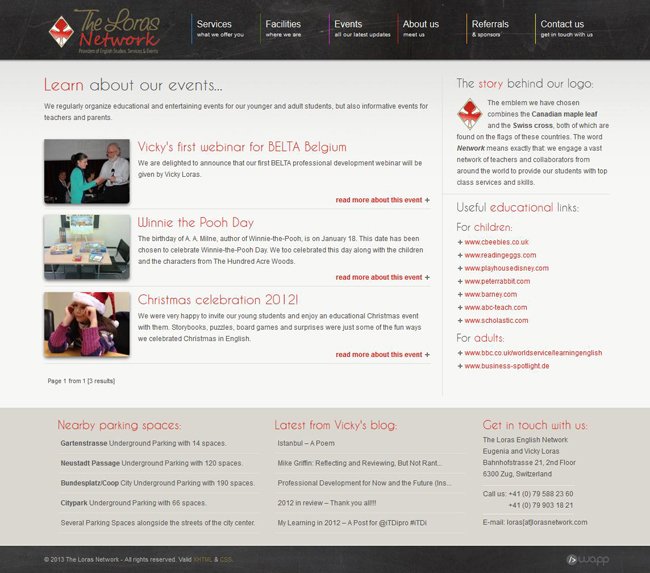### Detailed Caption for Screenshot

---

**The LORAS Network Website Screenshot**

At the top of the screenshot, the website header prominently displays "The LORAS Network" in bold, followed by a phonetic spelling "L-O-R-A-S." The main navigation menu features the following sections: "Services" (what we offer you), "Facilities" (where we are), "Events" (all our latest updates), "About Us" (meet us), "Referrals and Sponsors," and "Contact Us" (get in touch with us).

---

**Main Content Area**

The main content section begins with an announcement: 

**"Learn About Our Events"**

- **Regular Events:** This includes a brief description of the various events organized by The LORAS Network, highlighting educational and entertaining activities for both younger and adult students, as well as informative events for teachers and parents.

- **Vicky's First Webinar for BELTA Belgium:** The first professional development webinar by BELTA will be conducted by Vicky LORAS. The description is accompanied by a photo of an older man with a white beard handing a microphone to a woman, presumably Vicky LORAS.

- **Winnie the Pooh Day:** This section, next to an image of a table adorned with various items, mentions the celebration of A.A. Milne's birthday on January 18 by commemorating Winnie the Pooh Day with students and characters from the Hundred Acre Woods.

- **Christmas Celebration 2012:** A photograph of a woman wearing a Santa hat accompanies this segment. It describes a festive and educational Christmas event for young students, featuring storybooks, puzzles, board games, and surprises, all conducted in English.

**Right Side Bar**

- **The Story Behind Our Logo:** Describes the emblem combining the Canadian maple leaf and the Swiss cross, representing the origins and network of The LORAS Network. It emphasizes collaboration with teachers and professionals worldwide.

- **Useful Educational Links:** 
  - **For Children:** Links include websites like cbebies.co.uk, readingeggs.com, playhousedisney.com, peterrabbit.com, barney.com, abc-teach.com, and scholastic.com.
  - **For Adults:** Resources listed are bbc.co.uk/worldservice/learningenglish and business-spotlight.de.

---

**Nearby Parking Spaces:**

Detailed information about parking locations:
- **Gartenstrasse Underground Parking:** 14 spaces.
- **Neustadt Passage Underground Parking:** 120 spaces.
- **Bundesplatz/Co-op City Underground Parking:** 190 spaces.
- **City Park Underground Parking:** 66 spaces.
- **Street Parking:** Several spaces available in the city centre.

---

**Latest from Vicky's Blog:**

- **In Stambul, a Poem**
- **Mike Griffin:** Reflecting and reviewing but not ranting.
- **Professional Development for Now and the Future:** A 2012 review, expressions of gratitude.
- **My Learning in 2012:** A post for @tdipro, hashtag #itdi.

---

**Contact Information:**

- **The LORAS English Network:**
  - Address: Eugenia and Vicky Loras, Bahnhofstrasse 21, second floor, 6300 ZUG, Switzerland
  - Phone Numbers: +41 079 588 2360, +41 079 903 1821
  - Email: loras@lorasnetwork.com

**Copyright:** 2013 The LORAS Network, all rights reserved.

---

This detailed caption offers a comprehensive summary of the content and layout of the screenshot, covering the essential sections and their respective details.